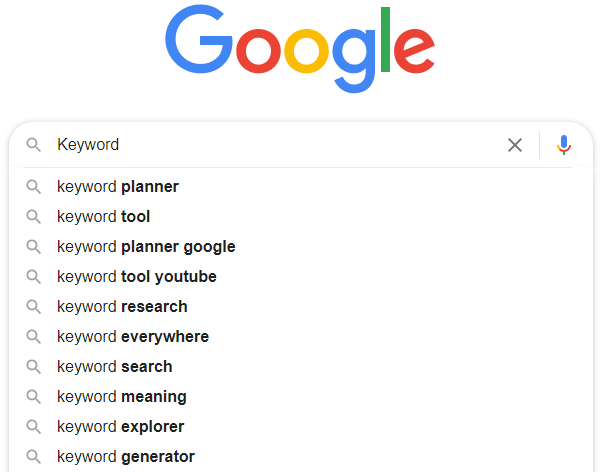The image depicts a Google search page. The background is predominantly white. At the top center sits the iconic Google logo, characterized by its vibrant colors: a capital 'G' in green, followed by a red 'o,' a yellow 'o,' a lowercase 'g' in blue, a green 'l,' and a red 'e.' Directly beneath the logo is the search bar, starting with a gray magnifying glass icon on the left side. Adjacent to the magnifying glass, the text inside the search bar reads "keyword" in black font. On the far right within the search bar are an 'X' symbol followed by a blue microphone icon, which has a red, yellow, and green base, indicating the voice search functionality.

Below the search bar is a thin, horizontal gray line extending across the width of the page. Underneath this line, aligned to the left, is a vertical list of search suggestions. Each suggestion is accompanied by a magnifying glass icon. The list of suggestions reads as follows: "keyword planner," "keyword tool," "keyword planner Google," "keyword tool YouTube," "keyword research," "keywords everywhere," "keyword search," "keyword meaning," "keyword explorer," and "keyword generator."